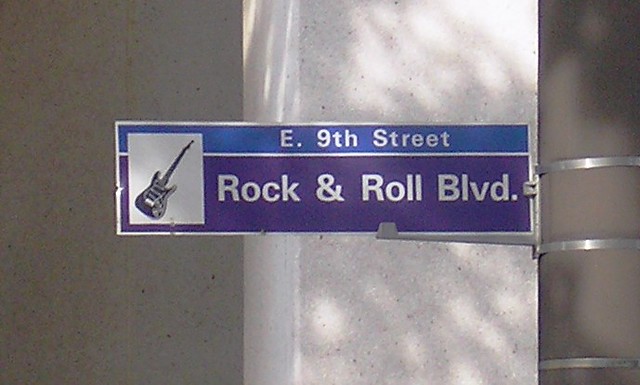The image captures a rectangular photograph of a street sign taken in an outdoor urban setting. The street sign prominently displays the text "E 9th Street" in white on a blue background, and "Rock and Roll Boulevard" in white on a purple background. To the left of the text, a black and gray electric guitar is depicted against a white square backdrop. The sign is affixed securely to a metal pole with metal rings, indicative of its robust installation. Behind the sign, a light gray wall can be seen, transitioning to a darker gray wall towards the left side of the image. The tight cropping of the photograph focuses closely on these detailed elements, emphasizing the vibrant colors and iconic representation of the guitar, which underscores the musical theme of the location.